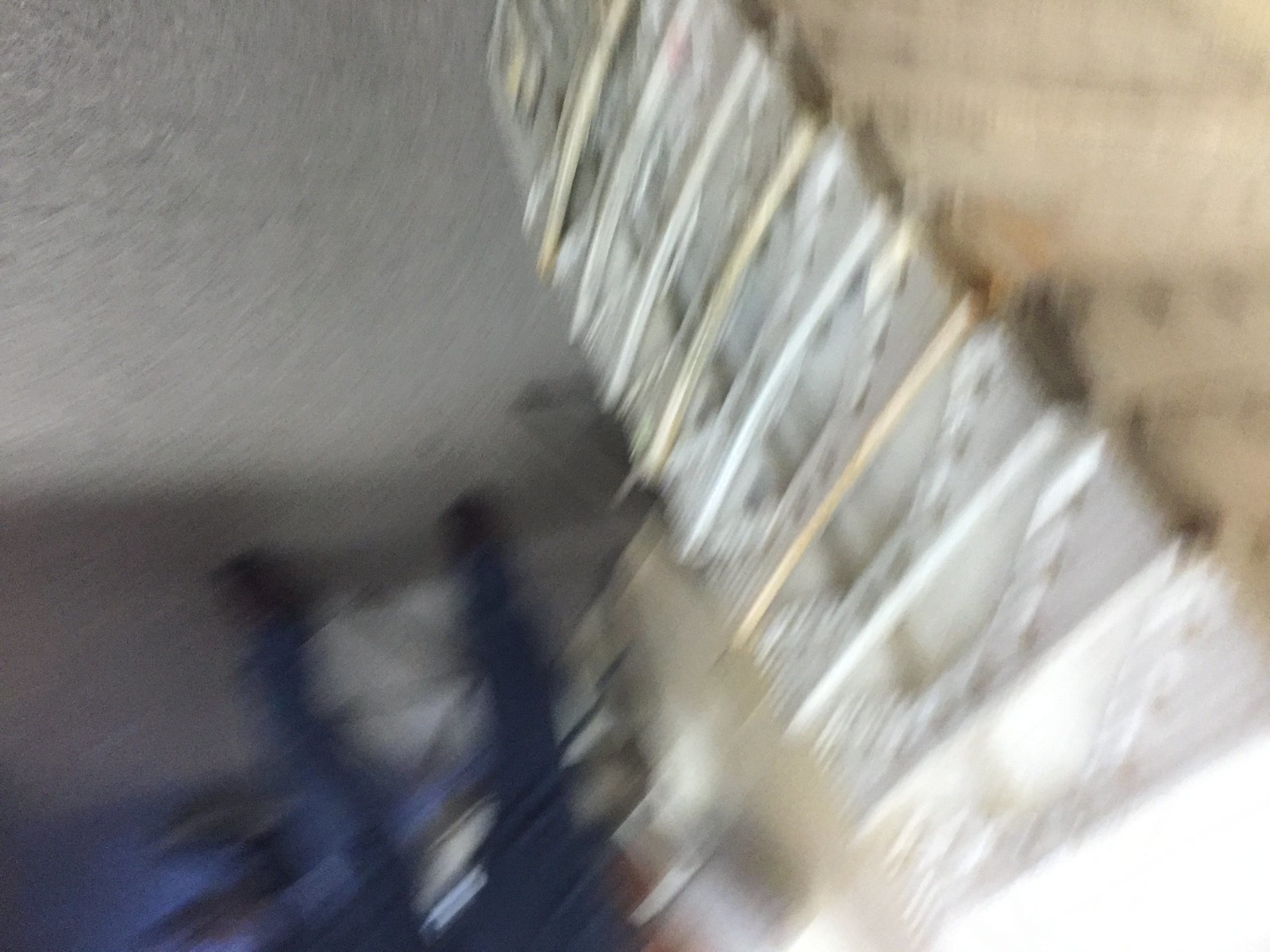This color photograph is heavily out of focus, resulting in a highly ambiguous image. On the right side of the photo, there appears to be a long, metallic rectangular shape, extending from the lower right-hand corner up towards the top center. This object may be the fretboard of an electric guitar or electric bass, characterized by its silverish hue and potential presence of strings and metallic crossbars. The left side of the image seems to show a gray ceiling in contrast with a darker gray wall, which possibly features two windows. Blue draperies, likely royal blue, frame these windows, adding a splash of color to the otherwise monochromatic scene.